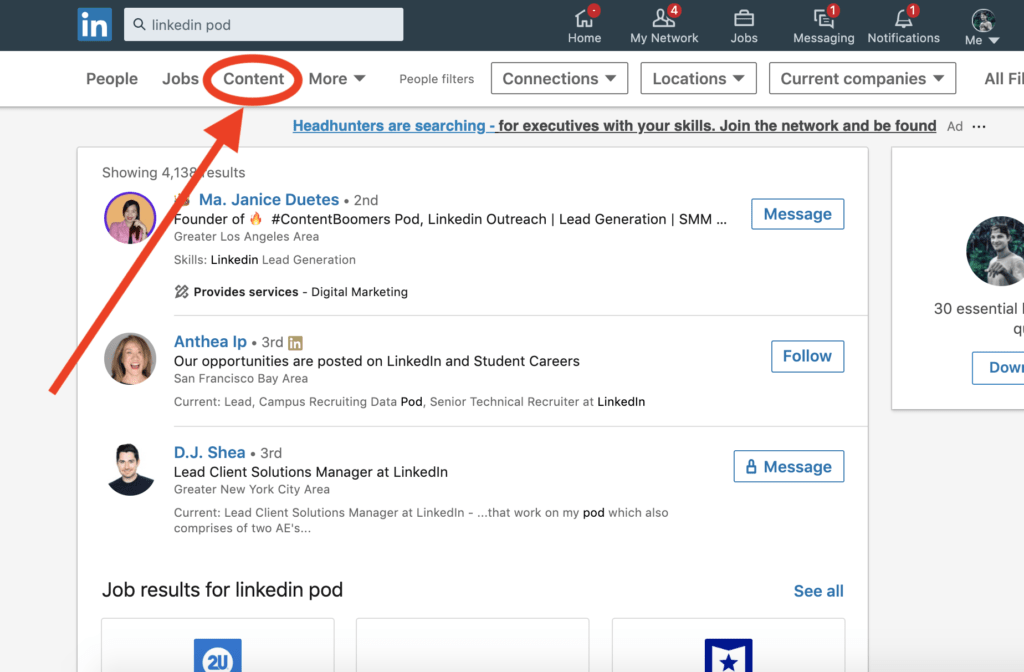This image displays a screenshot of a LinkedIn webpage. At the top, a black navigation bar spans the width of the screen, with a small blue box featuring the white letters "IN" on the far left. Adjacent to it is a white triangular area labeled "LinkedIn pod." The navigation menu includes icons and labels, all in white, for "Home," "My Network," "Jobs," "Messaging," "Notifications," and "Me," positioned towards the right-hand side.

Beneath this bar, additional tabs list options for "People," "Jobs," "Content," "More," along with filter categories such as "People filters," "Connections," "Locations," and "Current companies." There is some information on the screen's right side, which is partially cut off.

The central portion of the screen features a gray background with a prominent white box. At the top of this box, a message reads, "Headhunters are searching for executives with your skills, join the network and be found," followed by "AD..." 

Within this white box, there is a circular image of a woman whose name is obscured by a red arrow pointing upward to the tab labeled "Content," circled in red. Below her image, there is another picture of a woman named Athia, alongside a space titled "LP." Further down, a man's photo labeled "D. J. Shea" appears alongside more information about him.

At the very bottom of the image, it says "Job results for LinkedIn pod," with three white boxes partially cut off from the screen.